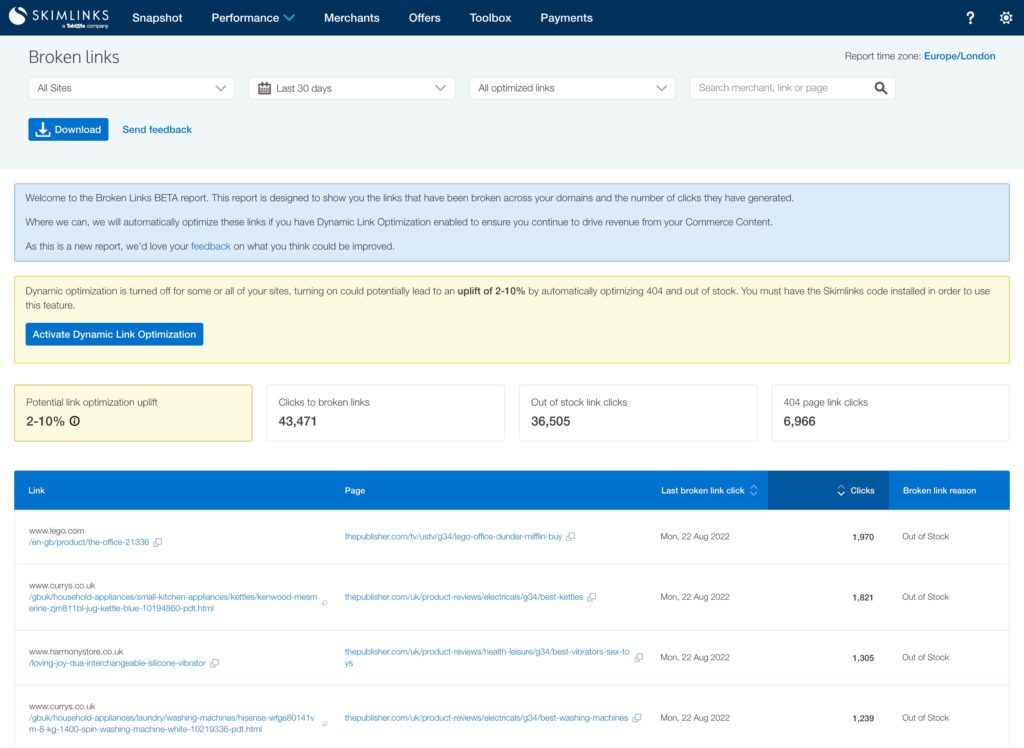In the image, the background is light blue with various elements layered on top, creating a complex interface. At the top, there is a darker blue square featuring a white circle with a blue checkmark. Inside this square, the words "SKIMLINKS," "SNAPSHOT PERFORMANCE," "MERCHANTS," "OFFERS," "TOOLBOX," and "PAYMENTS" are displayed, accompanied by a question mark and a gear icon.

Below this, the interface continues with the light blue background featuring broken link graphics. A search box labeled "ALL SITES" is centrally located, next to a blue "DOWNLOAD" button and a "SEND FEEDBACK" button. Directly below these, there are dropdown menus for "LAST 30 DAYS" and "ALL OPTIMIZED LINKS," as well as another search box labeled "SEARCH MERCHANT."

A large blue box labeled "BROKEN LINKS (BETA)" is also present. Next to it, a pink box labeled "DYNAMIC OPTIMIZATION" is shown as being turned off, with a blue button below it that says "ACTIVATE DYNAMIC LINK OPTIMIZATION." 

Another pink box shows a range of "2-10%" and includes a small black circle with a checkmark inside. Below this, various metrics are displayed, such as "GUIDE TO BROKEN LINKS: $43,472.00," "OUT OF STOCK CLICKS: $36,505.00," and another metric totaling "$6,966.00."

In the middle of the layout, a prominent blue box is labeled "LINK PAGE" and "LAST BROKEN LINE," accompanied by a blue "CHECK" button and an option to "RETAIN THE NAME." Below these, there's a list of additional items or settings.

Overall, this image presents a detailed dashboard interface, likely for managing and optimizing affiliate links, tracking performance metrics, and addressing broken links.